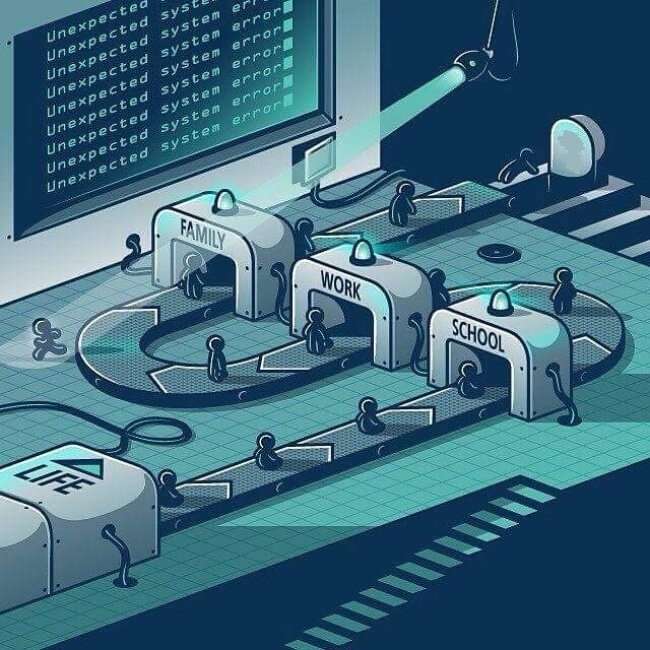The artwork depicted is a computer-generated illustration featuring various shades of blue, gray, and green. In the lower right corner, there are green stairs leading up to the scene. The central focus is a conveyor belt or pathway illustrating a cyclical journey of life stages: "Life," "School," "Work," and "Family," marked clearly on corresponding booths or structures. At the start, in the lower left corner, a bold white area reads "Life," from where small human figures embark on their journey. These figures progressively grow larger as they move through "School," "Work," and "Family," before collapsing face-first at the end of the path. Above this scene, an ominous, repetitive message, "Unexpected system error," is displayed on a video screen in the upper left corner. A spotlight shines on a single figure in the scene who appears to be running away, suggesting a moment of dissent or escape from the predetermined path. The backdrop of the scene includes gradients of blue and green, lending a somewhat surreal and digital aesthetic to the piece.